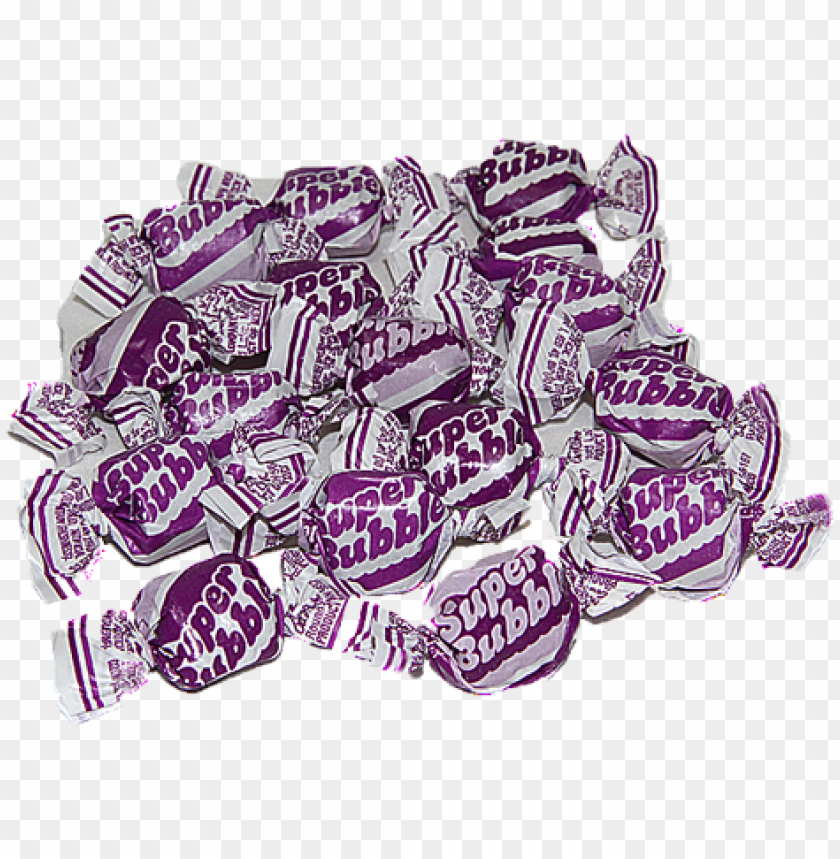The image features a neatly arranged pile of approximately 15-20 individually wrapped pieces of bubble gum, all labeled "Super Bubble." Each piece is ensconced in a paper wrapper with twisted ends, showcasing the text "Super Bubble" prominently in large white letters against a purple background, set on an additional white background. The background of the image displays a gray and white checkerboard pattern, indicating that the actual intended background is transparent. The gum pieces overlap each other and are centrally positioned within the image, creating a visually appealing mound of nostalgic candy. The predominant colors in the image are purple, white, gray, and off-white, suggesting a clean and digitally prepared photograph suitable for use as clipart on a website.